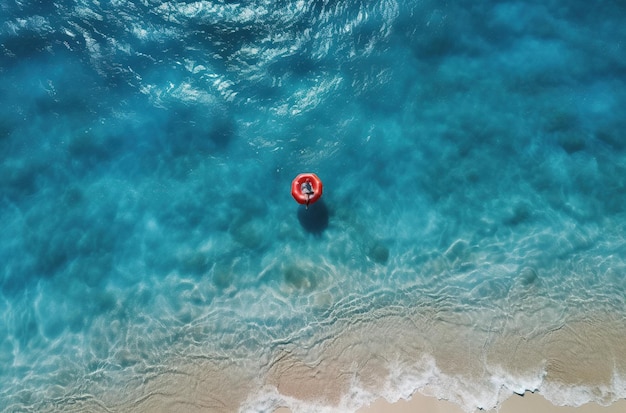The photograph, taken from an elevated perspective possibly by a drone or helicopter, captures a stunning coastal scene. The clear, blue-green waters stretch out below, gradually darkening towards the top of the image, hinting at deeper areas of the ocean or lake. The water is crystal clear, allowing visibility all the way to the sandy bottom. The shoreline at the bottom of the picture features light tan sand with gentle waves crashing in, creating a white foamy contrast against the beach. The bright sunlight enhances the natural beauty, reflecting off the water's surface. Dominating the center of the image is a small circular raft, red in color, with a person visibly lounging on it. This vivid red dot stands out against the serene blue backdrop, drawing the eye to the tranquil scene of someone floating close but not quite at the shore. The entire composition exudes a sense of calm and picturesque beauty on a sunny day.